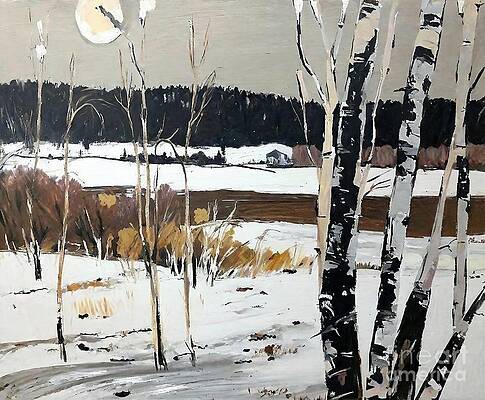This painting depicts a serene winter scene characterized by a muted palette of black, gray, white, and brown. The background features a dense, shadowy forest rendered in a dark silhouette against a cloudy gray sky, with a bright full moon illuminating the upper left corner. In front of the forest, layers of snow-covered fields stretch across the landscape, intersected by a central dirt road. Sparse, leafless trees and bushes—ranging in hues from red to yellow—line the road and provide depth to the scene. In the painting's right foreground, a close-up of a birch tree trunk, covered in snow, stretches from the bottom of the image upward. Further into the scene, a brown-toned body of water meanders through the snow, bordered by dead reeds and aqueous plants. A distant house and a brown fence add subtle details to the horizon, reinforcing the painting's tranquil, yet desolate winter ambiance.